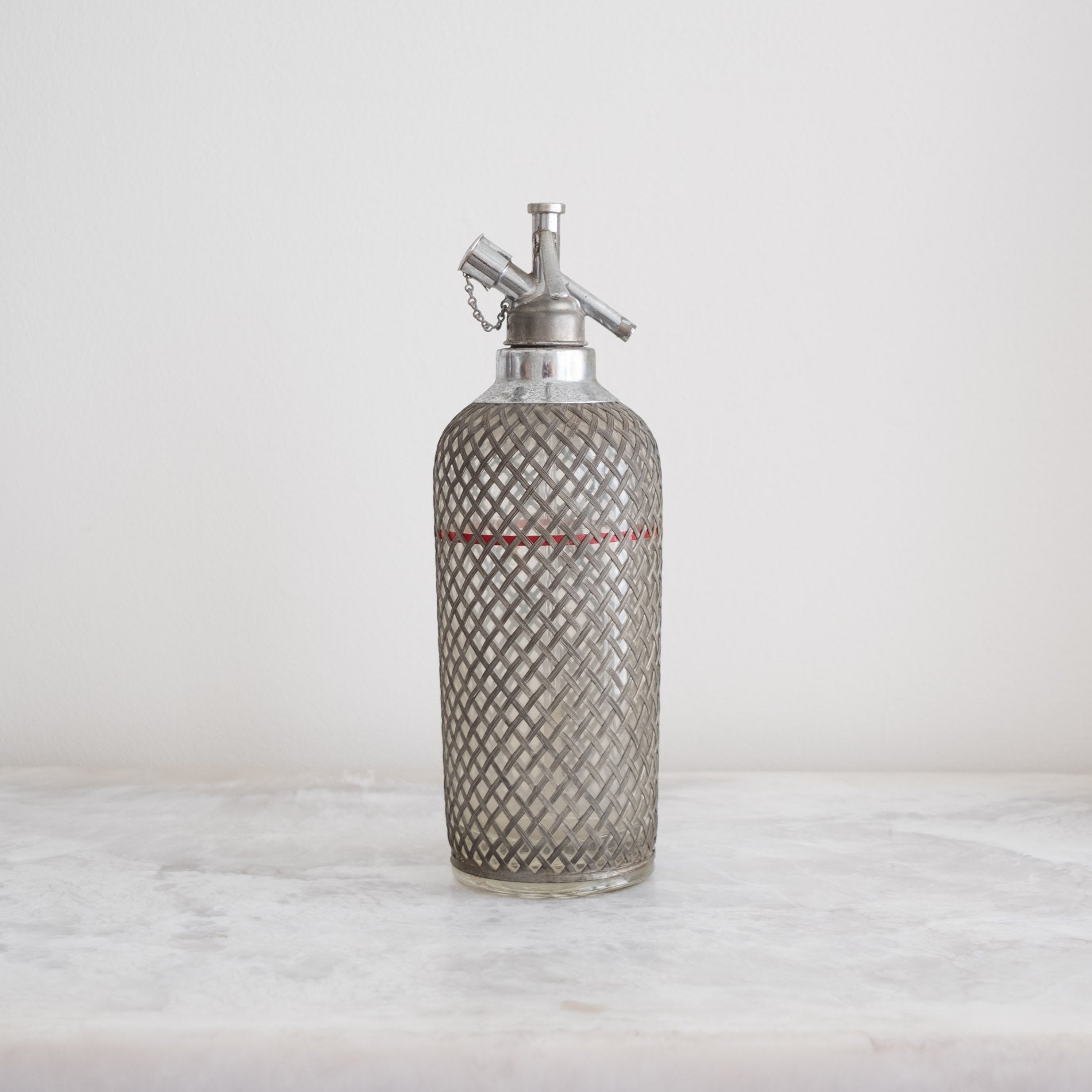The image displays a container that resembles a combination of a water bottle, a seltzer bottle, or a flask, featuring intricate detailing and a functional design. The cylindrical container stands approximately a foot to a foot and a half tall on a white-gray marble or granite countertop. The background showcases a light beige or off-white wall, offering a neutral and clean setting. The bottle itself features a checkered or woven pattern on its gray outer cover that partially reveals the glass or silver inner body. A distinctive bright red line accentuates the bottle about three-quarters of the way up, providing the only vibrant color in the otherwise monochromatic scene. The top of the bottle is equipped with a metallic, stainless steel sprayer or a unique closure mechanism, including a small cap or peg attached by a tiny chain. The overall image is centered on this elegantly designed container, emphasizing its detailed craftsmanship and the interplay of different textures and materials in a minimalist setting.